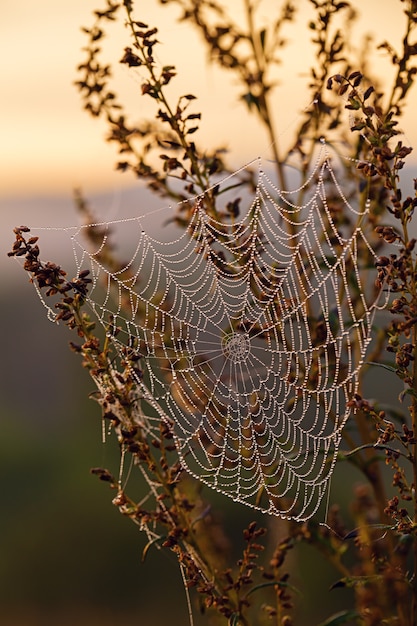In this close-up image, a plant with dark green, slender stems is prominently featured. The central focus of the plant is an intricately woven spiderweb, exhibiting a symmetric, circular shape and glowing in stark white. Although the spider itself is not visible, the delicate web stands out against the vibrant green backdrop. The background below is lush with greenery, while the center reveals hints of distant blue mountains. Above, the scene is kissed by soft hues of light yellow and light orange, suggesting either dawn or dusk. The background is artistically blurred and faded, providing a serene and dreamy contrast to the detailed foreground.